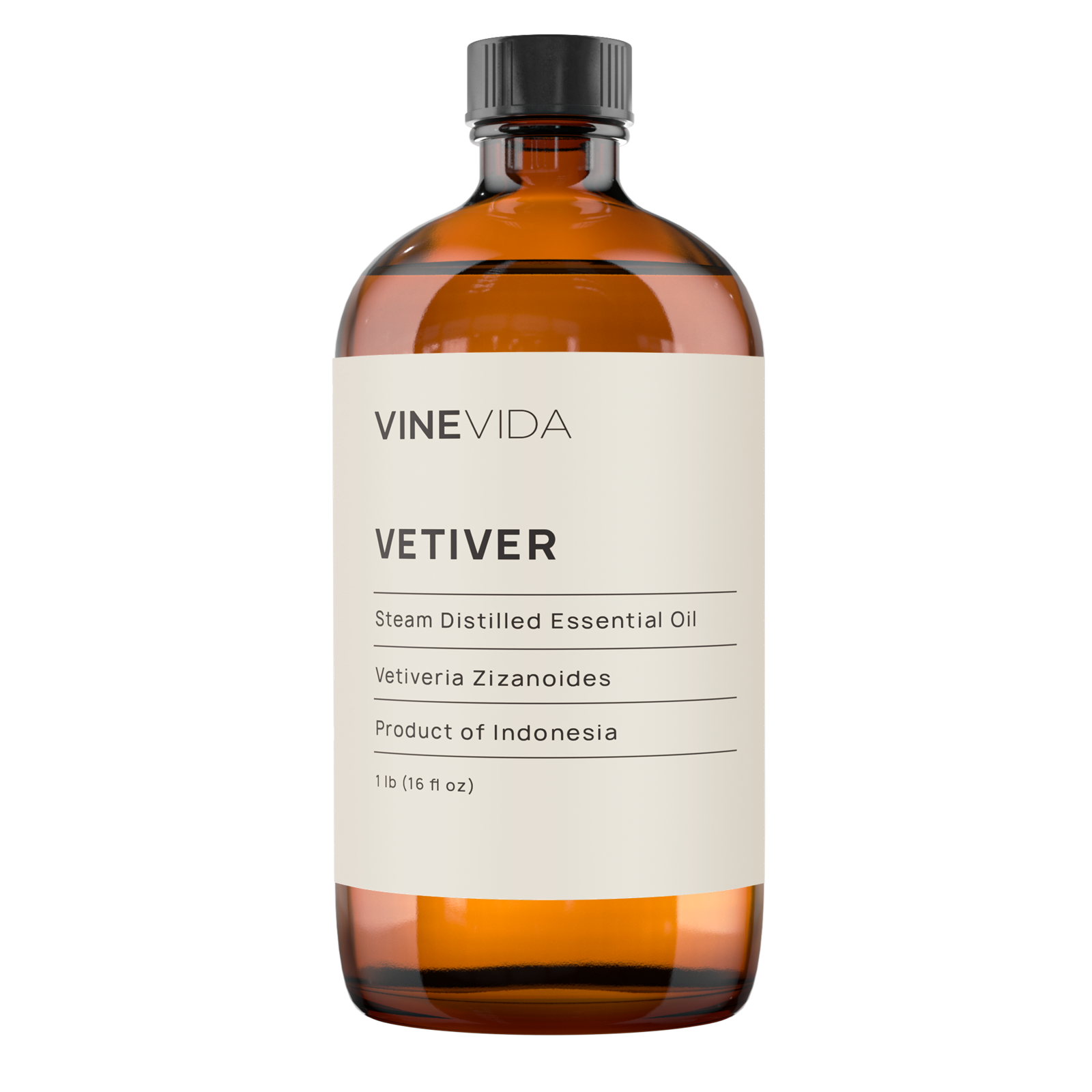The image is a close-up photograph of a modern apothecary bottle, isolated on a white background and placed on a flat white surface. The bottle is made of amber-brown glass and has a shiny finish, complemented by a black twist-off cap at the top. It features a wide, cream-colored label wrapped around its cylindrical body. The label is detailed with bold and narrow black text, all left-justified. At the top of the label, "Veen Vida" (or possibly "Vine Vida"), with "Veen" in bold sans serif lettering, is prominently displayed. Below this, the text "VETIVER" appears in all capital letters and bold. Underneath are several lines of descriptive text separated by narrow black horizontal lines: "steam distilled essential oil," "Vetiveria Zizanoides," "Product of Indonesia," and at the very bottom, smaller text reading "1 LB (16 FL OZ)."